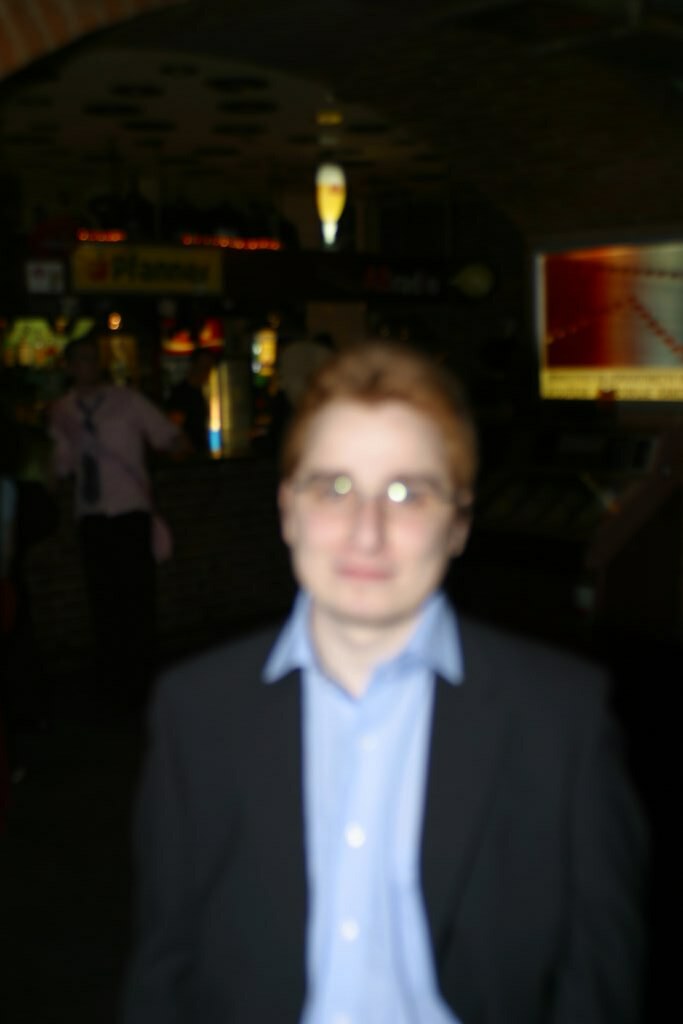A person with red hair and glasses, wearing a light blue collared shirt paired with a darker jacket, stands prominently at the forefront of the image. He appears to be in a dimly lit setting, possibly a street, studio, or a dark room. To his left, a second individual is standing, dressed in a white shirt and black tie, with black pants. This person also has a light-colored bag slung across his body. In the background, another man dressed in a black shirt can be seen looking toward the camera.